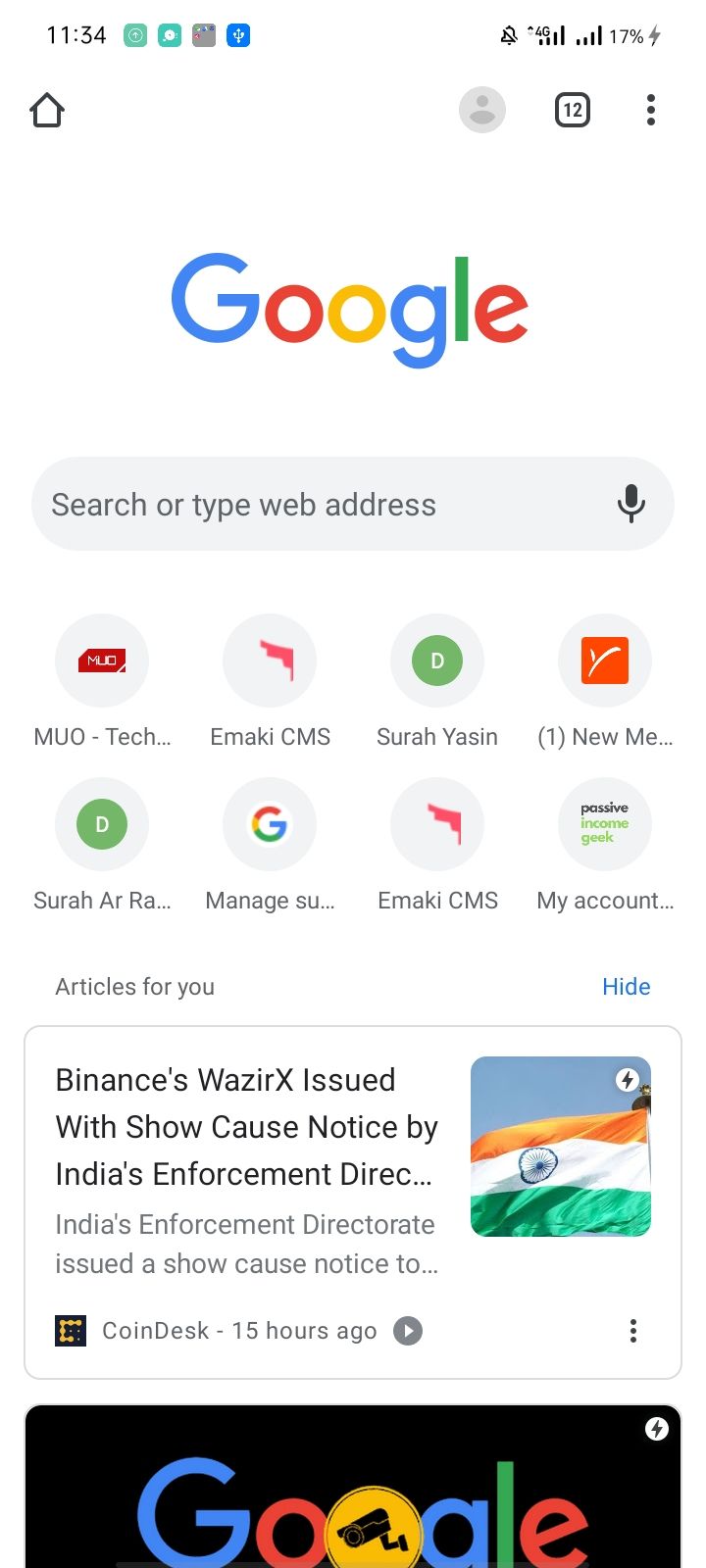The vertical image appears to be a screenshot taken from a smartphone. The upper left corner displays the current time, 11:34, along with several colorful icons. The background in this section is white, likely from a computer screen. 

In the upper right corner, various status indicators are visible, including a bell icon with a line through it, signal strength bars, a battery symbol showing 70% charged with a small lightning bolt indicating it's currently charging.

Below the time, there are several navigation icons: a house icon on the left, and a generic user profile circle, a box with the number 12, and three vertical dots symbolizing more options on the right.

At the center of the white background is the traditional Google logo, beneath which lies a gray search bar with the prompt "search or type web address" and a microphone icon on the right side.

Further down, there are partially visible text and icons related to content suggestions. These include names and terms like "M-U-O Tech", "Emaki CMS", "Sura Yassin", followed by a "(1 new M...)," "Sura R-Raw...", "Managesa..." and "my account..." The section is titled "Articles for you" with an option to "hide" highlighted in blue.

An article preview bordered by a gray box features the image of an Indian flag, followed by the article's heading, the author's name, and the publication time.

At the bottom of the image, there is a black bar with a Google icon.